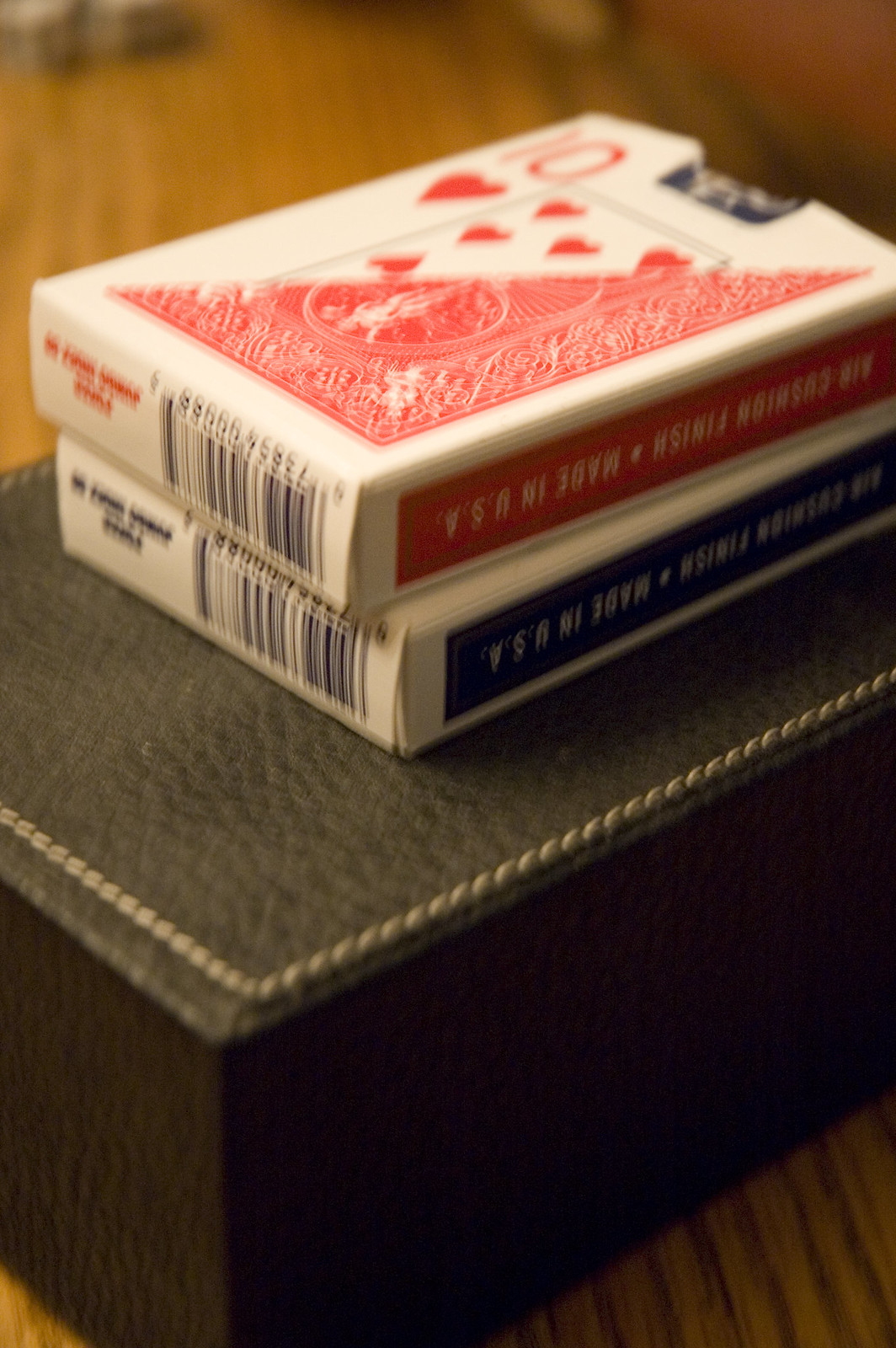This image features two decks of playing cards, one in a red box and the other in a blue box. Both decks display barcodes at the bottom, and the phrase "Made in USA" is printed along the sides. The red deck, clearly opened, rests on top of the blue deck, whose status cannot be determined. These decks are placed on a leather-bound item, possibly a journal or a photo album, which in turn rests on a wooden table. The setting includes a striped carpet with an orange background accented by black and red stripes. Additionally, the blue deck is situated on a green binder.